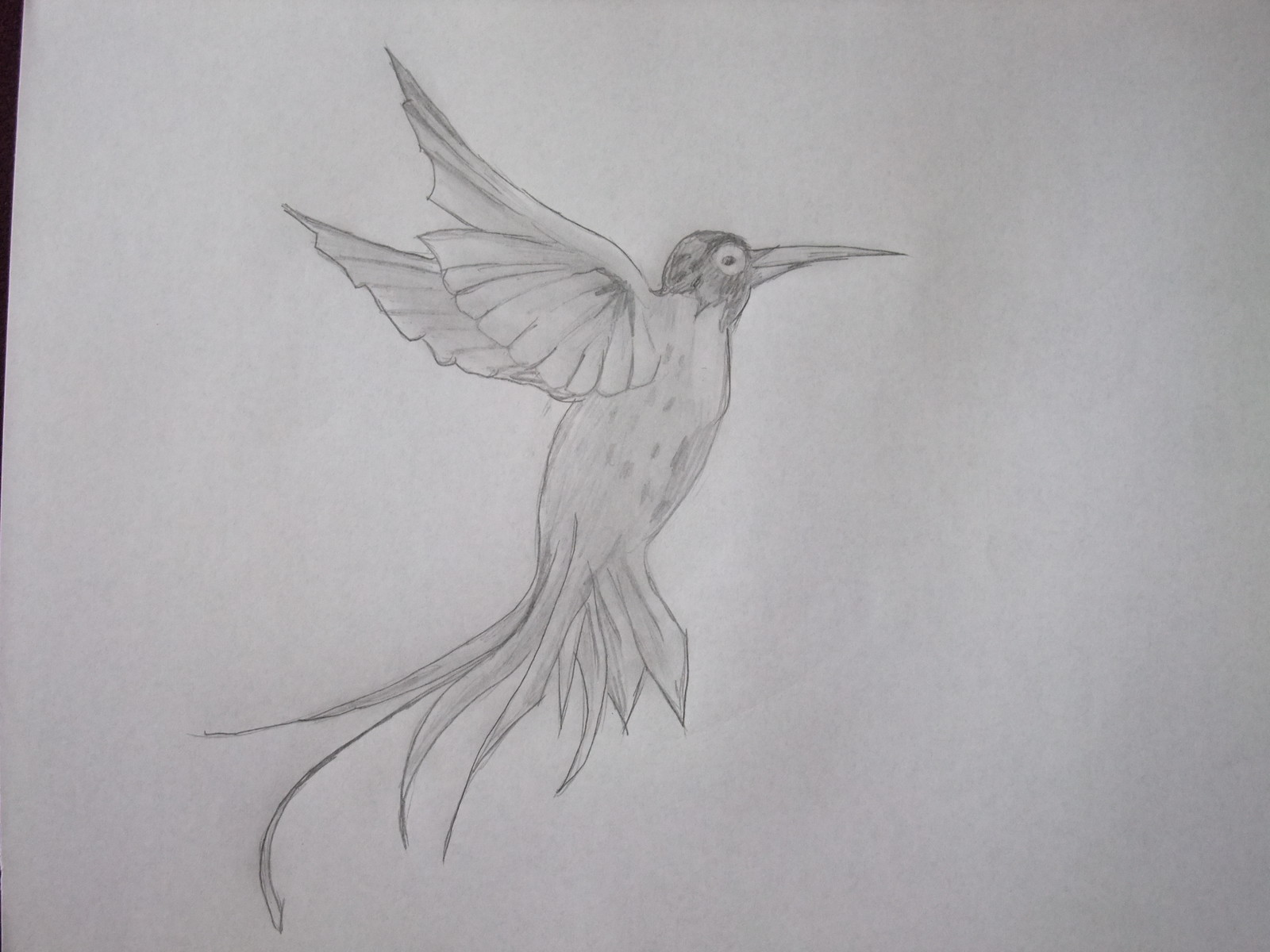This photograph captures a hand-drawn image on a slightly off-center sheet of white printer paper, revealing a small slice of a black background in the upper left corner. Rendered in gray pencil, the detailed sketch depicts a graceful bird, possibly a hummingbird, in mid-flight. The bird, oriented in profile facing right, showcases its long, pronounced beak, a distinctly darker head with a visible eye, and delicate spotting on its body. The wings, intricately detailed with visible individual lines, drape elegantly behind it, suggesting motion. The bird's body lowers into a flowing feathered tail that replaces the typical legs and feet, contributing to its elegant appearance. Light gray shadowing on the paper adds a subtle depth to the sketch, enhancing the bird's ethereal presence.